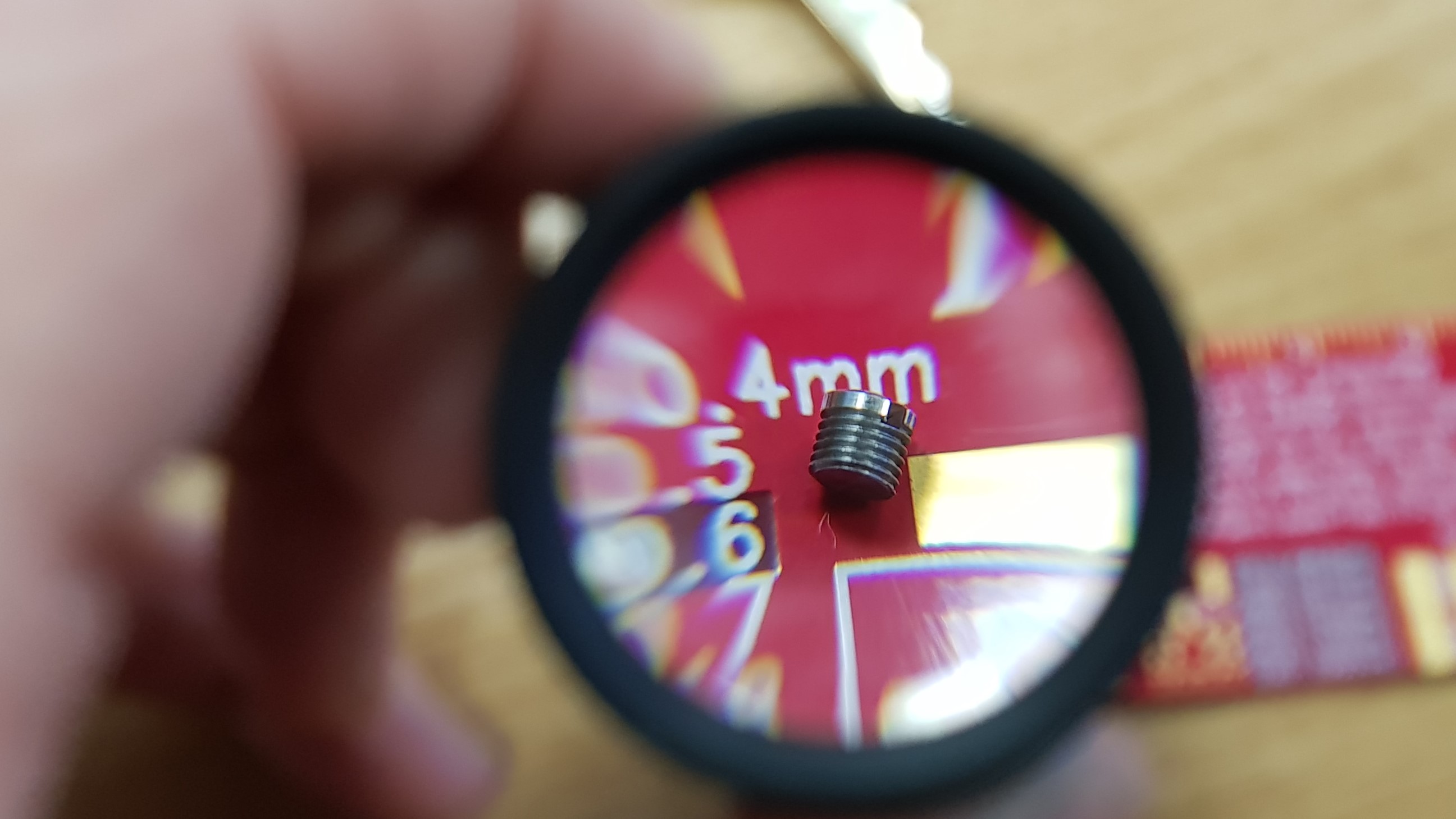In this detailed photograph, a human hand is seen holding a black-rimmed magnifying lens, which is closely focused on a very tiny silver screw or piece of metal hardware. The screw, notable for its rivets, is positioned against a red background featuring a scale marked in increments of millimeters (0.4, 0.5, 0.6, and 0.7). Though the surrounding details are blurred, the lens clearly magnifies the screw, making its intricate details vividly visible. The primary focus is on this minuscule screw, underscored by the precise measurements displayed in the background, with the overall scene capturing the precision of the magnification setup.